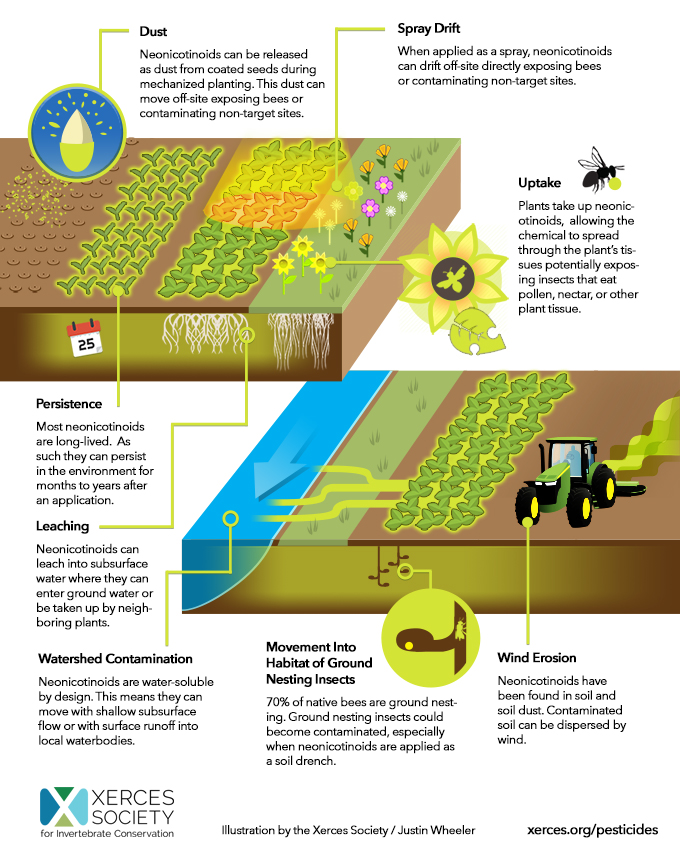This diagram, likely extracted from an educational brochure by the Xerces Society for Invertebrate Conservation and illustrated by Justin Wheeler, visually depicts the impact of pesticides on farmland using bright, colorful cartoon images. The diagram showcases fields of crops and flowers, featuring layers of soil and plants. Detailed annotations describe various aspects of pesticide interaction, such as dust, spray drift, uptake, persistence, leaching, watershed contamination, wind erosion, and the movement of pollutants into the habitats of ground-nesting insects. A green tractor is also prominently featured in one of the cutaway views, adding a cute and relatable element to the illustration. Additionally, there is a logo at the bottom – a white 'X' set against blue and green triangles – along with the website xerces.org/pesticides, indicating it is an authoritative source on environmental conservation issues. This diagram is vividly informative, aimed at raising awareness about the implications of pesticide use in agriculture.